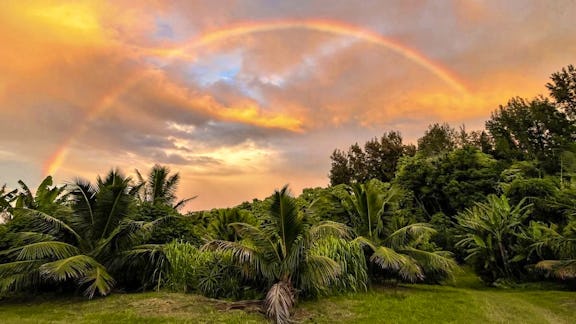This photograph captures a serene outdoor setting at sunset, showcasing a sprawling tropical landscape. In the foreground, a manicured, vibrant green lawn stretches across the bottom of the image. Rising above the grass, lush tropical plants and bushes are adorned with large leaves and palm fronds, creating a dense, verdant backdrop that transitions into taller trees ascending on the right side of the frame. The sky above is an exquisite blend of colors, with hues of orange, yellow, and pink painting a breathtaking sunset canvas. The clouds, particularly in the top left corner, are tinged with bright yellows, adding a luminous touch to the scene. Dominating the sky is a striking rainbow, arching gracefully from the bottom left to the top right, its faint yet distinct bands of red, yellow, green, and blue visible against the colorful sunset. The rainbow, while thin, spans impressively across the scene, adding a magical element to the tropical paradise.